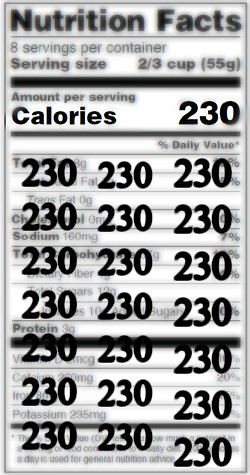A white portrait-oriented nutrition label is displayed against a white background. The label, originally handwritten in black ink, has the number "230" superimposed in bold, dark font above the photograph. The number "230" appears in rows of three and spans eight rows in total, indicating 230 calories per serving. The label details that there are eight servings per container, with each serving size being two-thirds of a cup.